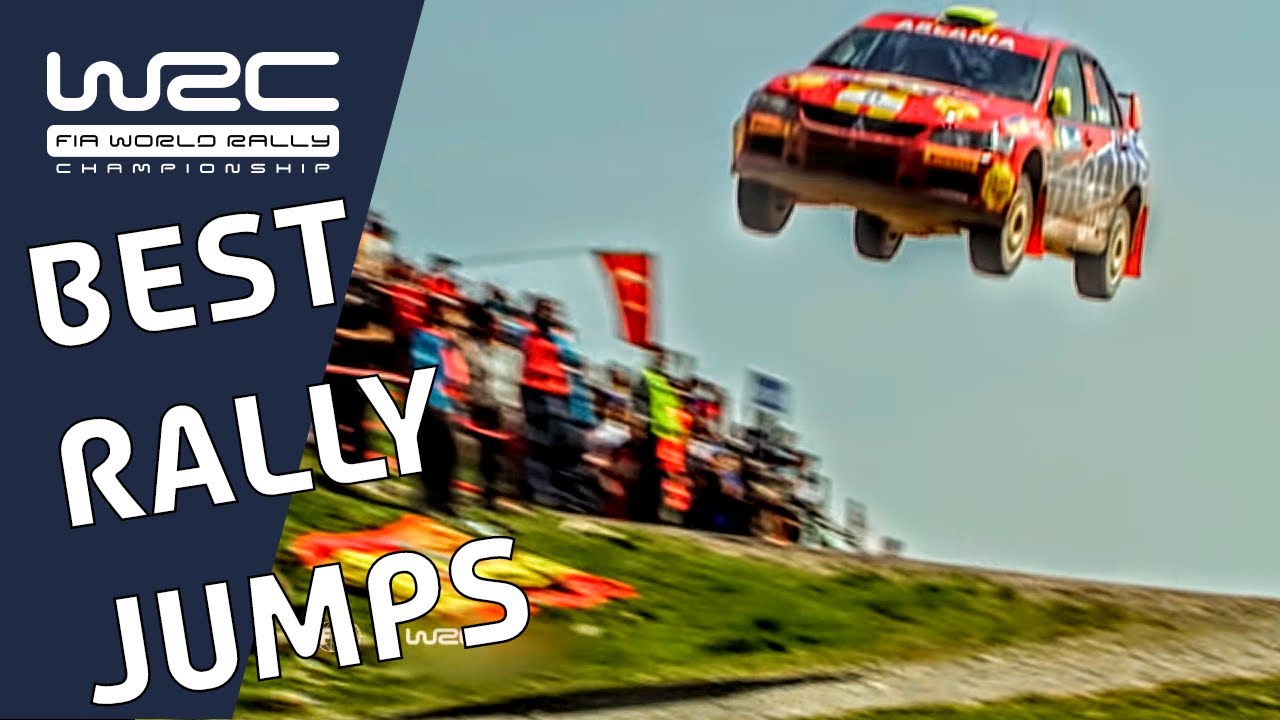This captivating photograph captures an intense moment in the WRC FIA World Rally Championship, showcasing one of the Best Rally Jumps. The eye-catching red rally car, adorned with a blue and white Mentos advertisement and Arania spelled on the front, soars through the air several feet off the ground. Its dynamic motion is emphasized by the slight blur, indicating its high speed as it approaches the photographer. Accents of yellow and orange on the boxy, early 90s-style car add to the vibrancy of the scene. On the left side of the image, a navy blue banner displays "Best Rally Jumps WRC FIA World Rally Championship" in bold white letters. Below the airborne car, green grass is visible, while a group of spectators stands on a hill, waving red flags and watching the thrilling moment unfold. Additional red and yellow flags lie directly underneath the car, adding to the scene's colorful and exhilarating atmosphere.